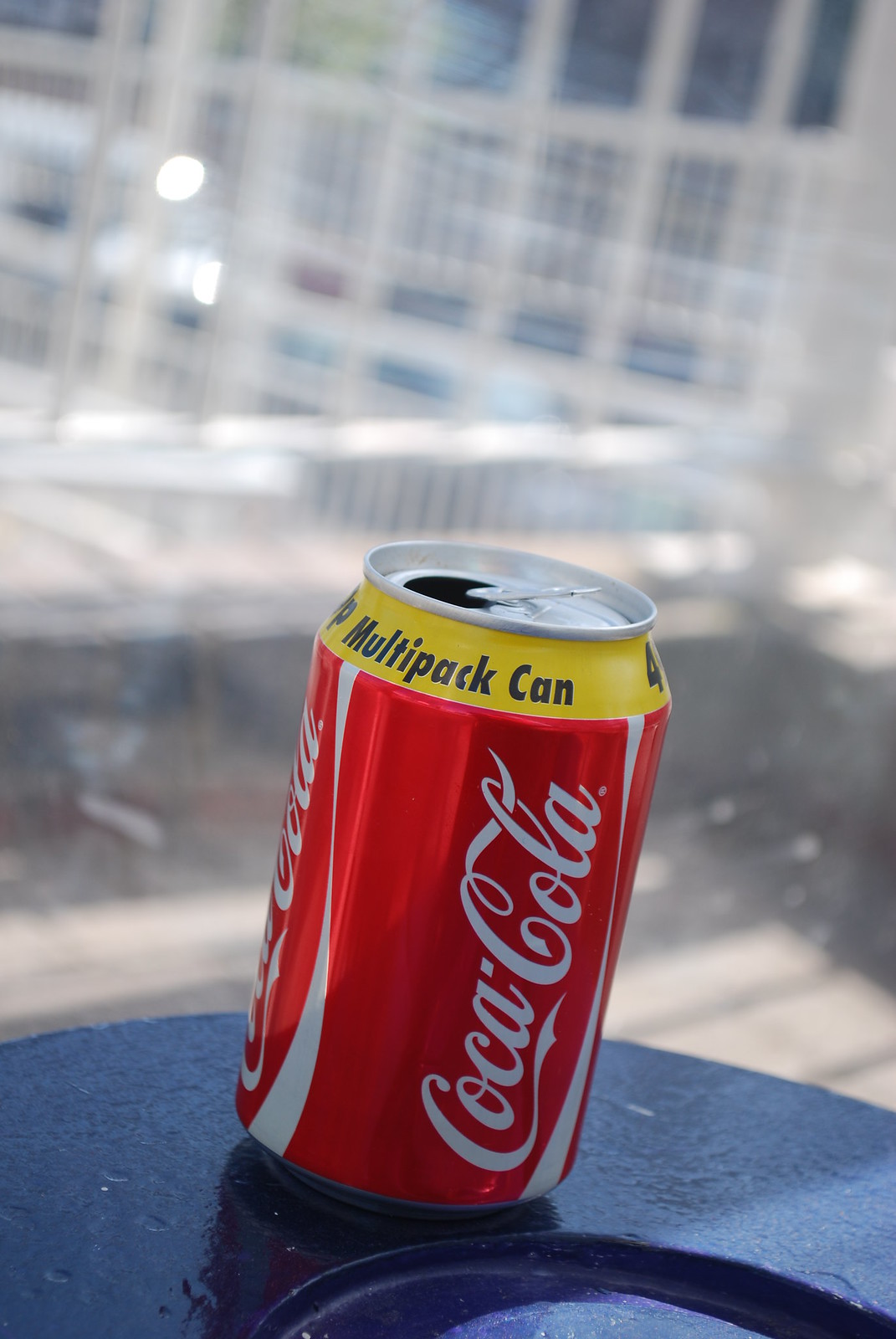The image is a vertically-oriented photograph, likely indoor but strongly illuminated by sunlight streaming through a large, blurred window or possibly a fence with white wooden frames, creating a cross-pattern effect in the background. At the bottom of the image, occupying roughly a quarter of the vertical space, is the edge of a shiny blue, metallic-looking plate. Atop this surface sits an aluminum, mini-can of Coca-Cola, distinguished by its traditional red body and white cursive logo. The can features a yellow banner at the top with "multi-pack can" printed in black, indicating it comes from a pack of cans.